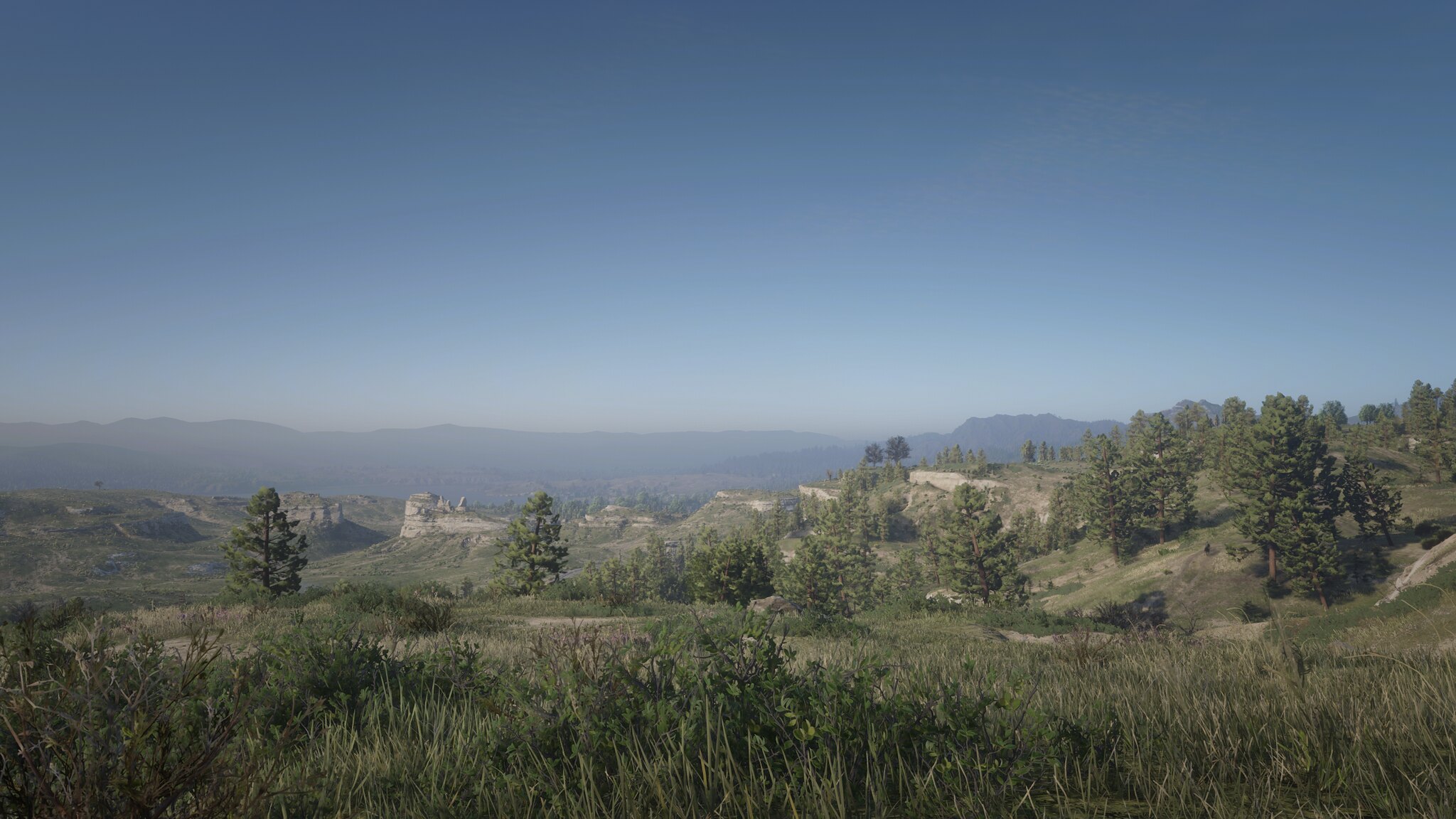A breathtaking outdoor landscape unfolds in this photograph, captivated under a vibrant blue sky. Toward the horizon, a gentle white haze subtly blends with the azure expanse, suggesting the warmth of the sun. Majestic mountains loom in the distance, their rugged peaks colored in gradient shades of gray and black.

The scene is dotted with scattered evergreen trees, standing individually or in sparse clusters, emphasizing the openness of the environment. The trees, distinct in their natural resilience, add a refreshing patch of green to the otherwise muted palette.

The ground is a textured mosaic of rocky outcrops and sandy patches, with hues of gray intertwined with tinges of yellow. Brown, coarse grass covers the ground in irregular patches, hinting at the arid conditions of the terrain. Scattered bushes add to the diversity of the vegetation, completing the composition of this serene, untouched landscape. No fauna is present, making the viewer's focus entirely on the stark beauty of the natural scenery.